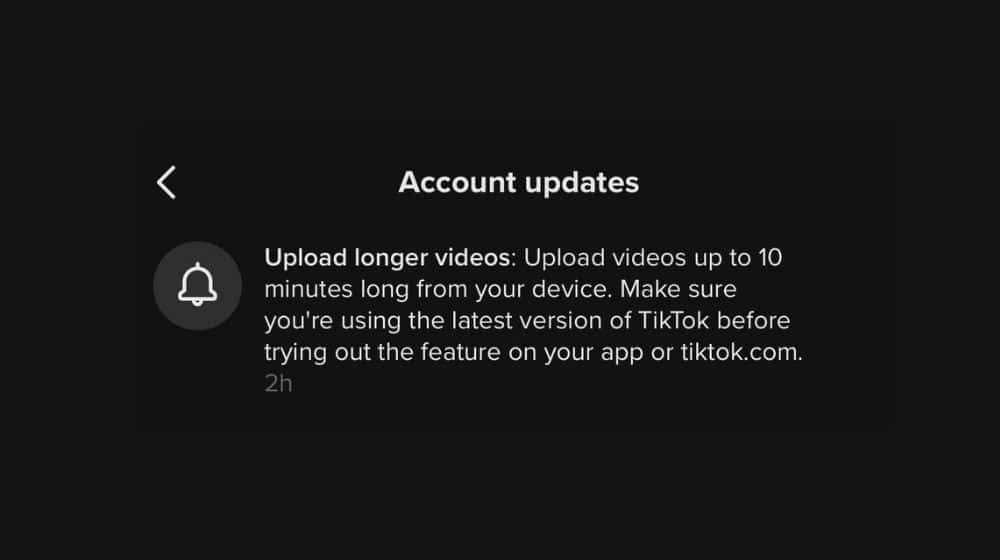The image displays an update message from TikTok against a stark black background. At the top center, the bold white text reads "Account Updates." Positioned to the left is a white arrow pointing left. Centrally located in the screenshot, there's a prominent bell icon within a lighter black circle, featuring a white bell in its center. Below this icon, the main message is clear and concise: "Upload longer videos" appears in bold white text. The message instructs users: "Upload videos up to 10 minutes long from your device. Make sure you're using the latest version of TikTok before trying out the feature on your app or tiktok.com." In the bottom left corner, it notes that the message was sent two hours prior to when the screenshot was taken. The "Account Updates" heading stands out in large, bold letters, while "Upload longer videos" is slightly smaller but equally bold.